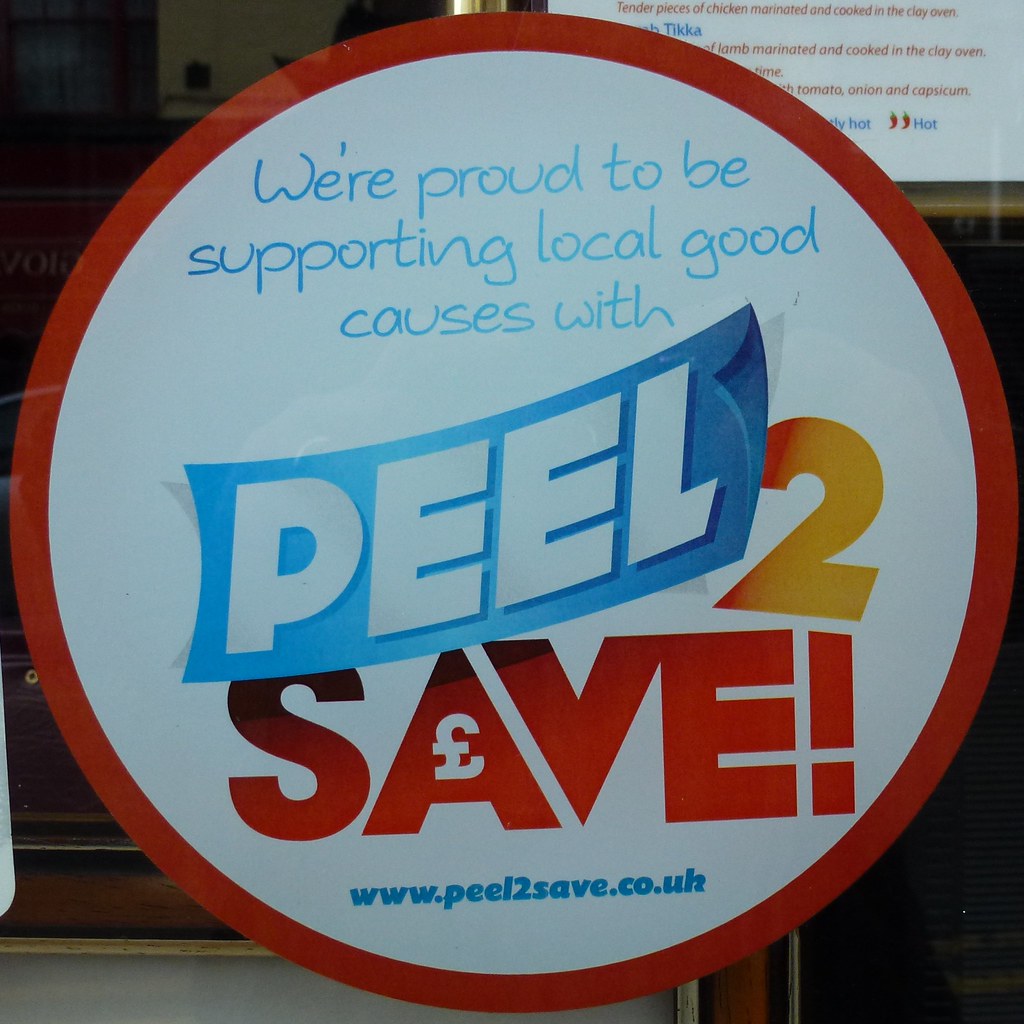The image shows a promotional sign prominently displayed outside a grocery store, featuring a circular design with a red border and a white background. At the top of the circle, there is blue handwritten text that reads, "We're proud to be supporting local good causes with." Below this, in the center, a large white text on a blue background boldly states "Peel," with the right edge of the word appearing as if it is being peeled up. An orange number "2" is positioned next to the word "Peel." Beneath this, in large red letters, is the word "Save," with the letter "A" replaced by a pound sign (£) and an accompanying exclamation point. At the bottom of the sign, there is a website URL in blue text: "www.peel2save.co.uk." In the background, faintly visible, is what appears to be part of a menu on a whiteboard with red text.